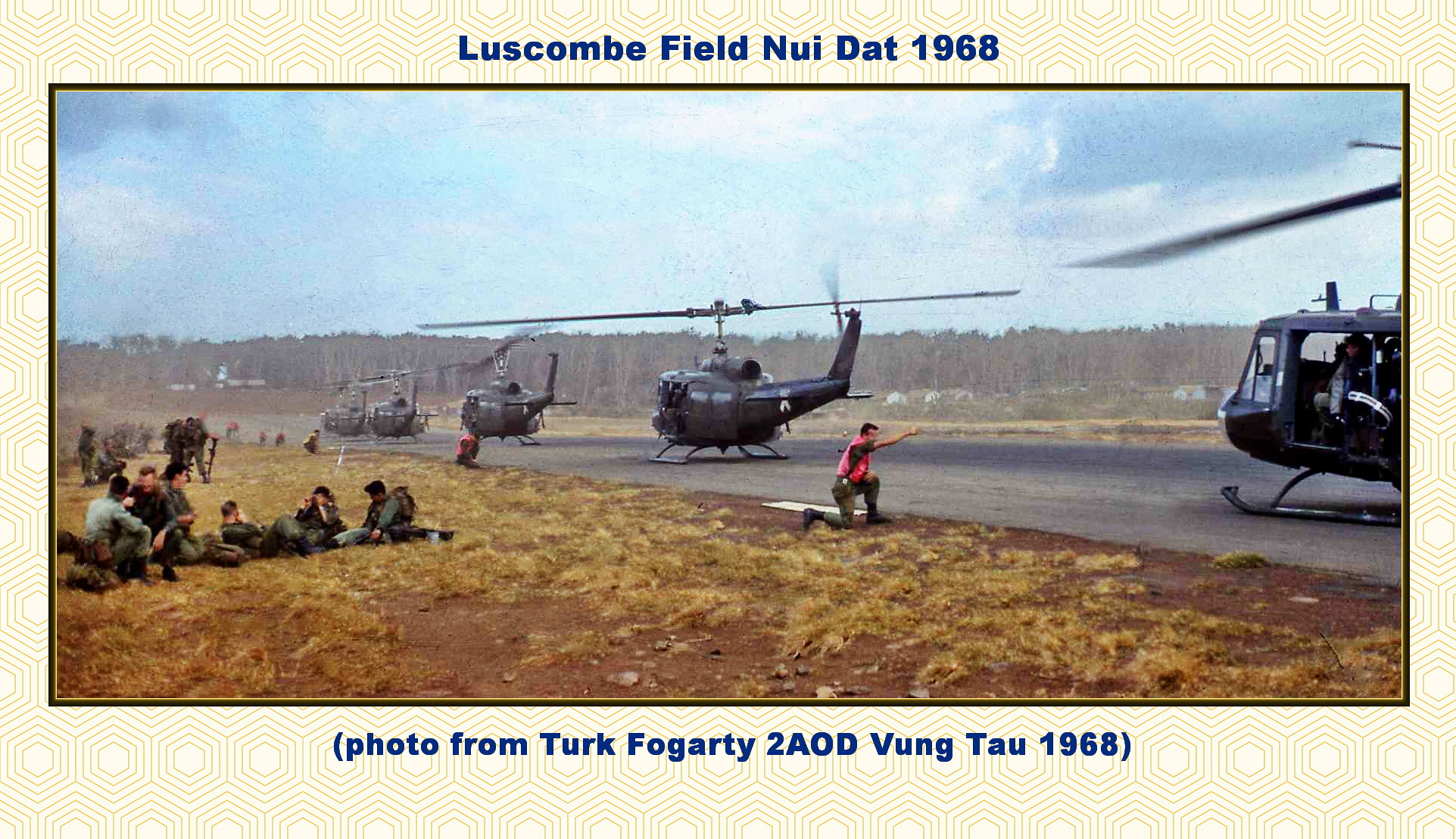This full-color photograph from 1968 depicts a scene from Luscombe Field, Nguyen Dat, Vietnam. In a narrow band of pavement at center stage, five helicopters are parked single file. The overcast daytime sky casts a muted light over the setting. Dominating the foreground, a man in a bright red or orange vest kneels beside the pavement, extending his right arm towards the helicopters as if directing them. Surrounding him in the patchy grass and dirt field to the left, several soldiers dressed in green army fatigues are either sitting or standing in small groups. The background reveals a dense crop of trees and additional grassy areas, creating a sense of depth. The photograph is bordered by a cream and blue frame, with text at the top reading "Luscombe Field, 1968," and at the bottom, "Photo from Turk Fogarty to AOD Vung Tau, 1968."